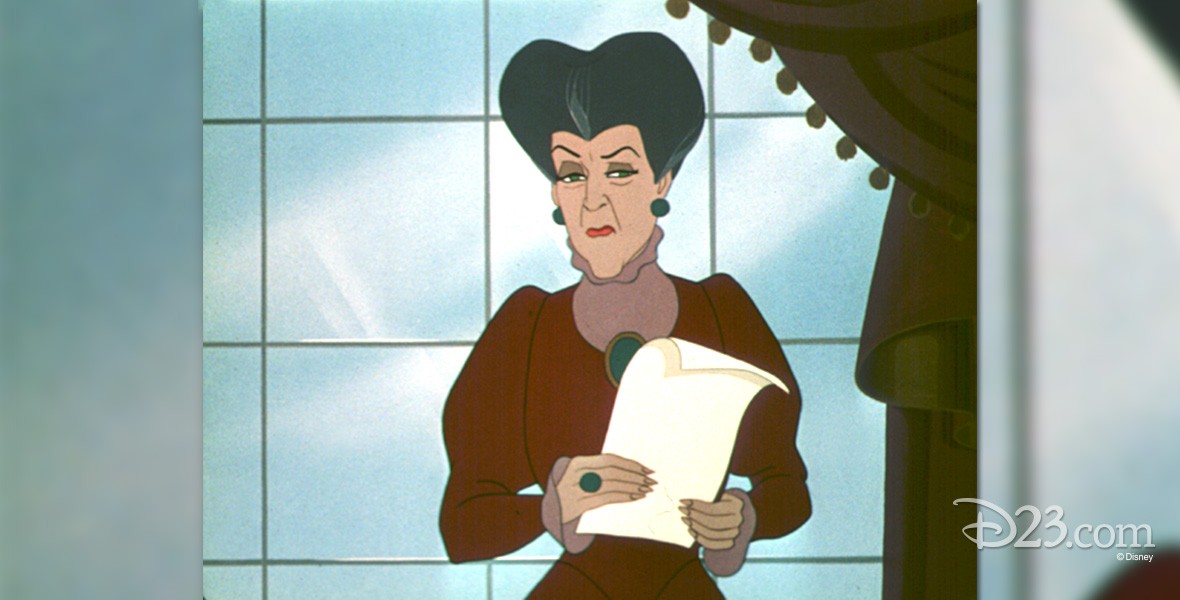This horizontally aligned rectangular cartoon image, with no visible border, features a detailed depiction of Lady Tremaine, Cinderella’s stepmother from the classic Disney animated movie “Cinderella,” likely sourced from d23.com, with a small copyright notice in the lower right corner indicating Disney’s ownership. Lady Tremaine is portrayed as an older woman with very tall, short hair that is blackish-gray. She is wearing dark green, round earrings and a matching dark green pendant. Her long-sleeve dress is dark brown with bulky-looking upper arms, complemented by a circular green ring on her finger. She is holding a white sheet of paper that curves at the top and has a serious, almost disgusted expression, with green eyes, brown eye shadow, and curvy black eyebrows. In the background, there is a large square window with dark brown curtains on the right and a gray wall on the left. The scene captures her displeasure, possibly in the moment when she reads the notice inviting every eligible woman to the prince’s ball.